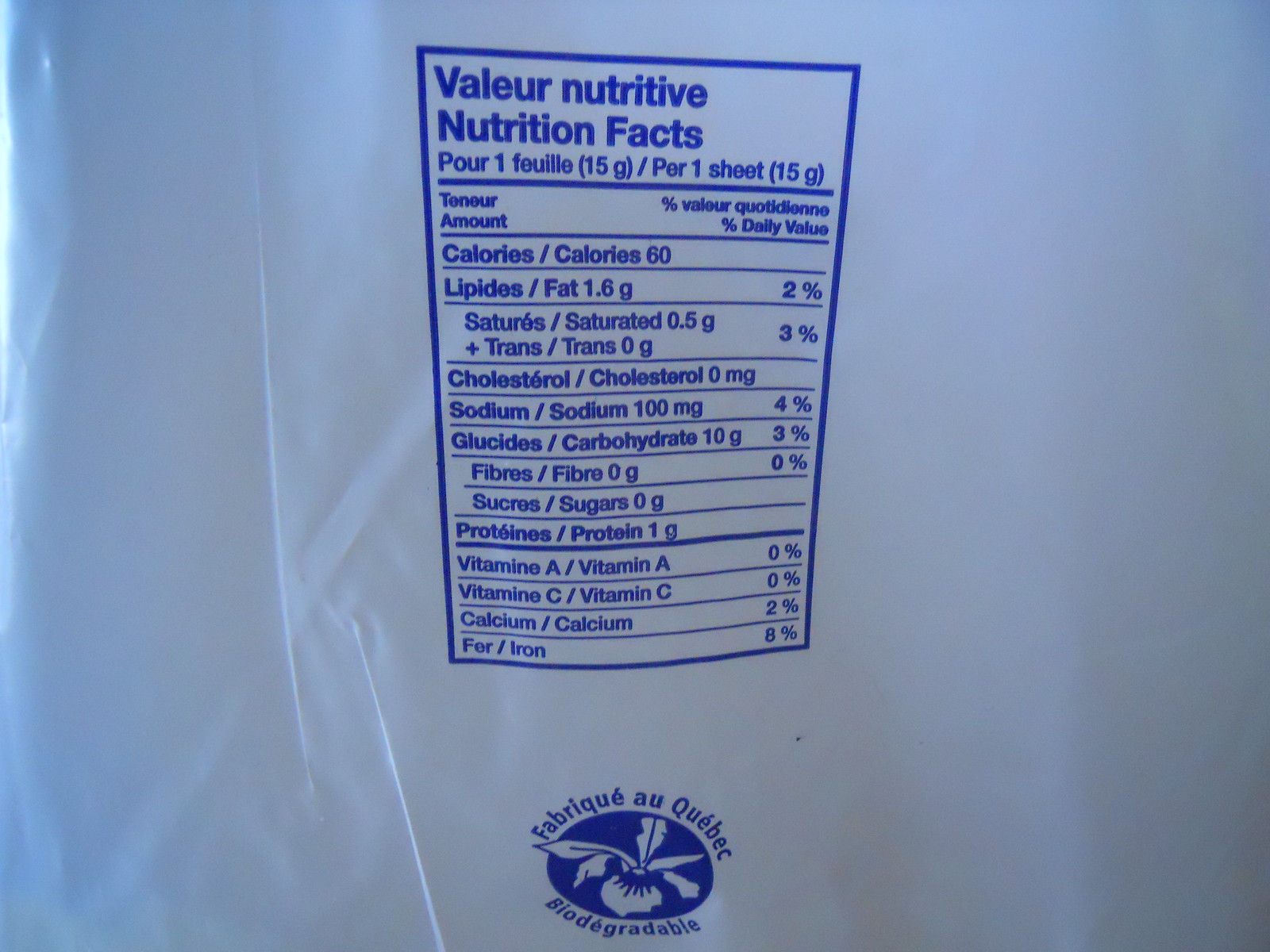This photograph displays a bilingual Nutritional Facts label, presented in both French and English. The label retains the standard rectangular format, clearly itemizing nutritional information per a 15-gram serving. It details essential data such as calories, fats, cholesterol, sodium, carbohydrates, fiber, sugar, proteins, vitamin A, vitamin C, and calcium. At the bottom of the label, there's a notable logo consisting of an image of a rapper, accompanied by the text "Fabriqué au Québec," indicating that the product was made in Quebec. Additionally, there is mention that the packaging is biodegradable plastic, emphasizing its environmentally-friendly aspect. The bilingual nature of the label ensures comprehensive understanding for both French and English-speaking consumers.